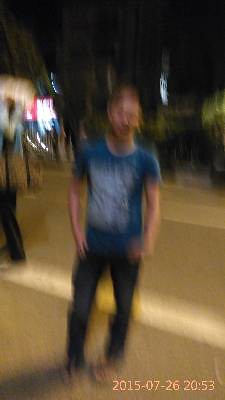A blurred nighttime image captures a young Caucasian man standing on a roadway or pavement, intersected by a white line running diagonally from the lower right to the upper left. The background is enveloped in darkness, punctuated by dim, colored lights and faint outlines of other people, suggesting he might have been walking along the street when the photo was taken. The man, sporting short brown hair, wears a round-neck, short-sleeved t-shirt adorned with a large, light-colored design dominating the front. He pairs this with black jeans or pants. His hands rest casually by his sides, close to his pockets.